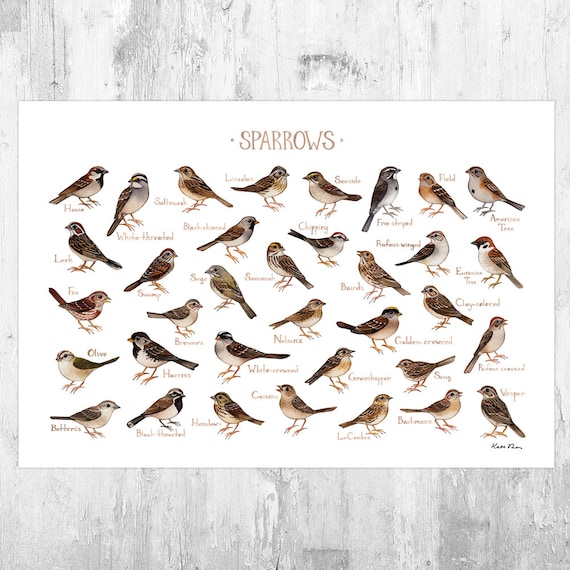The photo captures a detailed poster pinned against a light gray wooden wall, showcasing a diverse array of sparrows. The poster, titled "Sparrows" prominently at the top, features a white background adorned with meticulously drawn illustrations of about 36 different types of sparrows. These birds are primarily brown with subtle variations in shades, such as hints of black, white, orange, and even charcoal gray. The sparrows are depicted standing, each accompanied by small, difficult-to-read labels identifying their species. Notable names that are slightly legible include the house sparrow, white-throated sparrow, grasshopper sparrow, olive sparrow, and seaside sparrow. In the bottom right corner of the poster, there is a black signature of the artist.